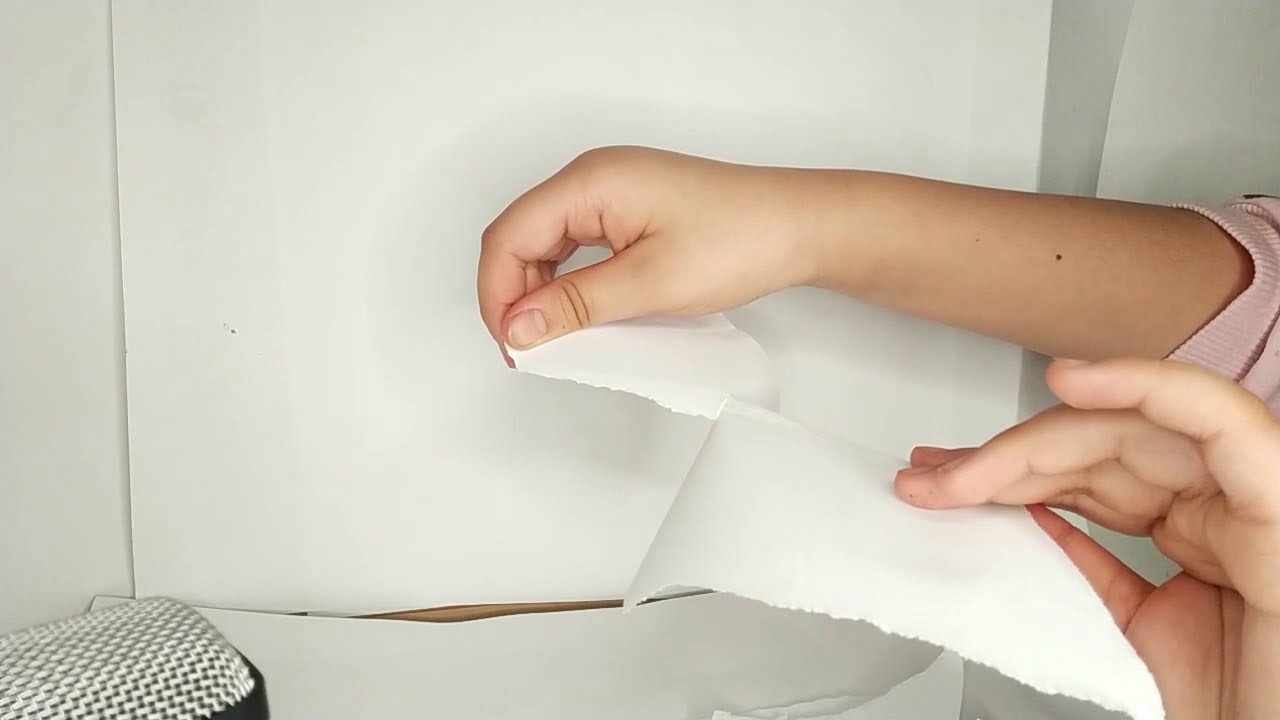The photograph captures a close-up scene of a person's hands in the act of tearing a white piece of paper. The individual, who appears to be wearing a light pink sweatshirt or short-sleeved shirt, has one piece of the paper grasped in their right hand and the other piece in their left hand, with the tear happening in the middle. The person's hands, which are slightly chubby and of a lighter skin complexion, are in motion, emphasizing the dynamic action of ripping the paper. The background is predominantly white, possibly featuring white wallpaper or numerous strips of white paper, some of which are already torn. In the lower left corner, part of a purse and a microphone can be seen, adding context to the setting. The scene is well-lit, suggesting natural light, which adds to the bright and clear ambiance of the image.